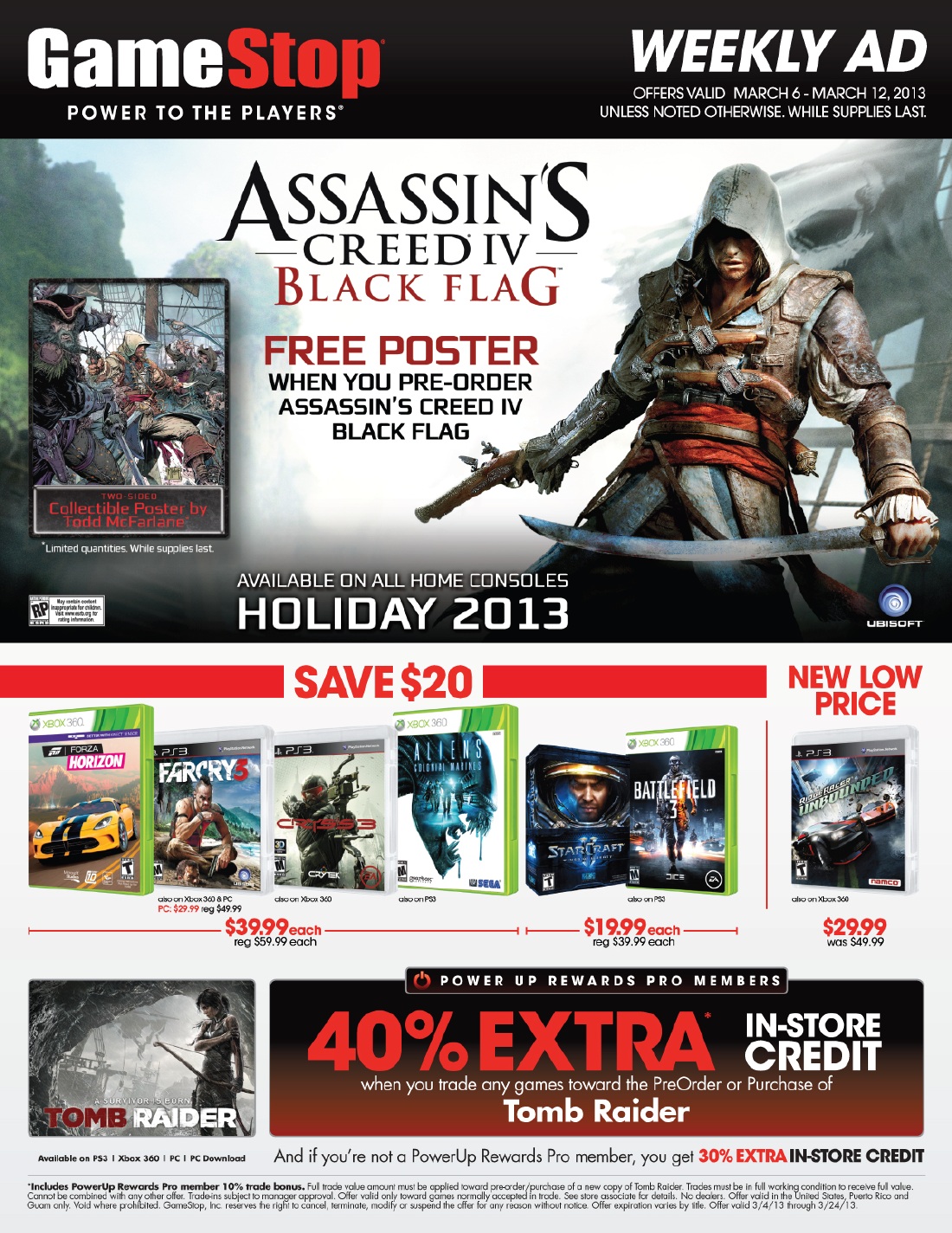Caption: 

"This detailed GameStop poster prominently features the brand's logo and tagline, 'Power to the Players', positioned in the top left corner. Adjacent to this, on the right, the text announces the 'Weekly Ad' with offers valid from March 6th to March 12th, 2013. Dominating the center of the poster is an eye-catching promotional image for 'Assassin's Creed IV: Black Flag', highlighting a pre-order special that includes an exclusive poster. The artwork depicts a formidable assassin clad in a grayish cloak, wielding a sword in his left hand and a Derringer pistol in his right, set against a backdrop evocative of the Age of Sail. Below this centerpiece, the poster advertises a $20 savings on a selection of popular games. Titles on offer include Forza Horizon, Far Cry 3, Crysis 3, Battlefield 3, and the latest Tomb Raider, alongside various coupons and attractive discounts."